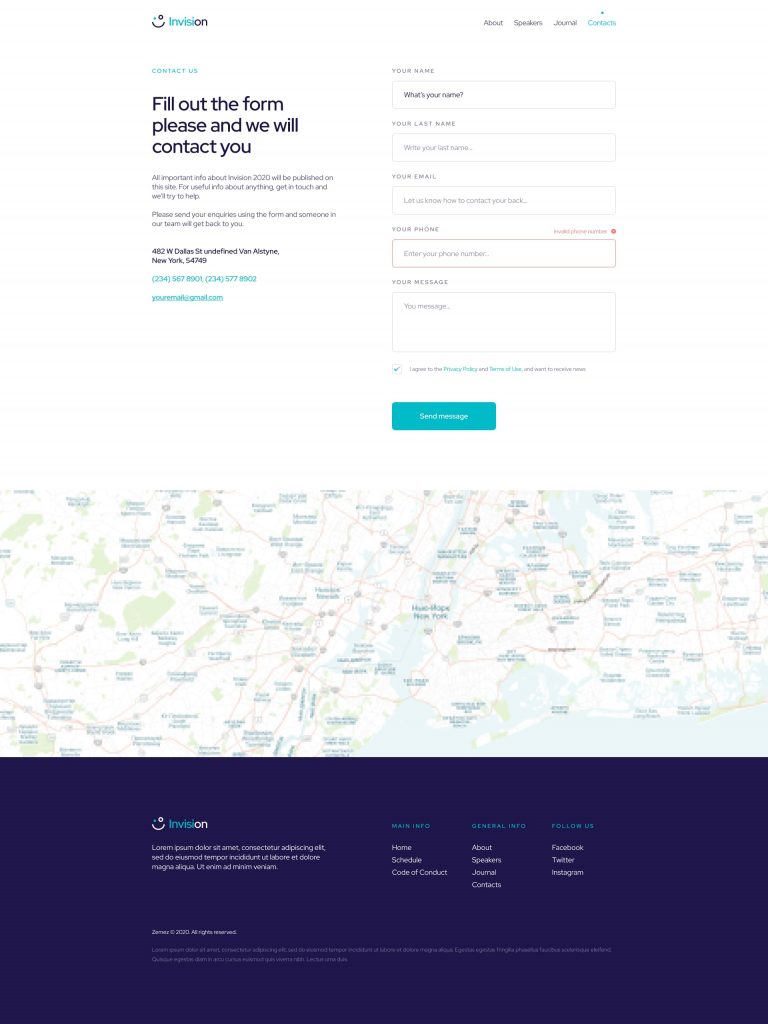This is an image from the company InVision displayed against a white background. In the top left corner, the word "InVision" appears, with "In" in light blue ink and "Vision" in dark blue ink. To the right, there are several navigation options: "About," "Speakers," "June," and a category that might be "Contacts." Beneath these, in tiny light blue letters, is the phrase "Contact Us." Below this is a bold navy blue statement: "Fill out the form, please, and we will contact you." 

Following this text, a smaller, unreadable address is listed. To the right of this information, there are several input boxes for sending a message: "Your First Name," "Your Last Name," "Your Email," "Your Phone," and "Your Message." A light blue turquoise box labeled "Send Message" is present for submitting the form. 

Beneath the form is an image of a map with annotations, though the text and region details are too small to discern. At the very bottom of the image is a thick blue ribbon spanning the width of the page, with the word "Envision" in white text. Underneath, there are various clickable categories for further navigation, including: "Home," "Code of Conduct," "About," "Speakers," "June," "Contact Us," "Facebook," "Twitter," and "Instagram."